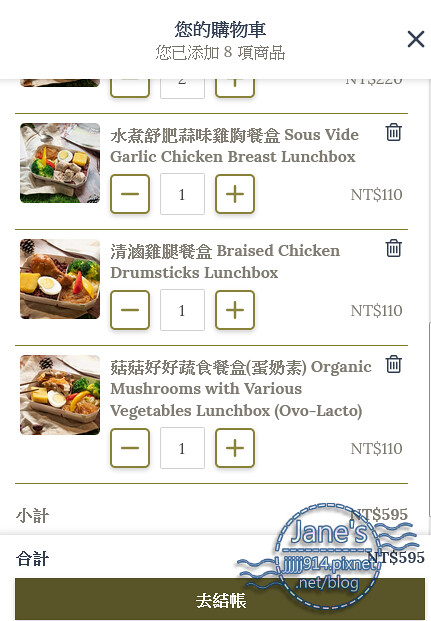The image depicts a user interface for an online food menu, most likely from a Chinese restaurant. The background is predominantly white, with distinct sections demarcated by dark gray lines, each containing a picture of food on the left. Adjacent to each image, there are the dish's name in both Asian characters and English, spanning one or two lines. The menu lists a variety of options, such as "Garlic Chicken Breast Lunchbox" priced at NT$110, "Braised Chicken Drumsticks Lunchbox" also at NT$110, and "Organic Mushrooms with Various Vegetables Lunchbox (Ovo-lacto)" for NT$110. At the bottom of the interface, there's a logo or icon labeled "Jane's," accompanied by the text "Jane's Circle with squiggles" and a URL "janes.j914picsnet.net/blog." The setup appears very user-friendly, featuring plus and minus boxes to adjust the quantity of each item. The text is mostly in Chinese or potentially Japanese, suggesting the target audience for this menu.